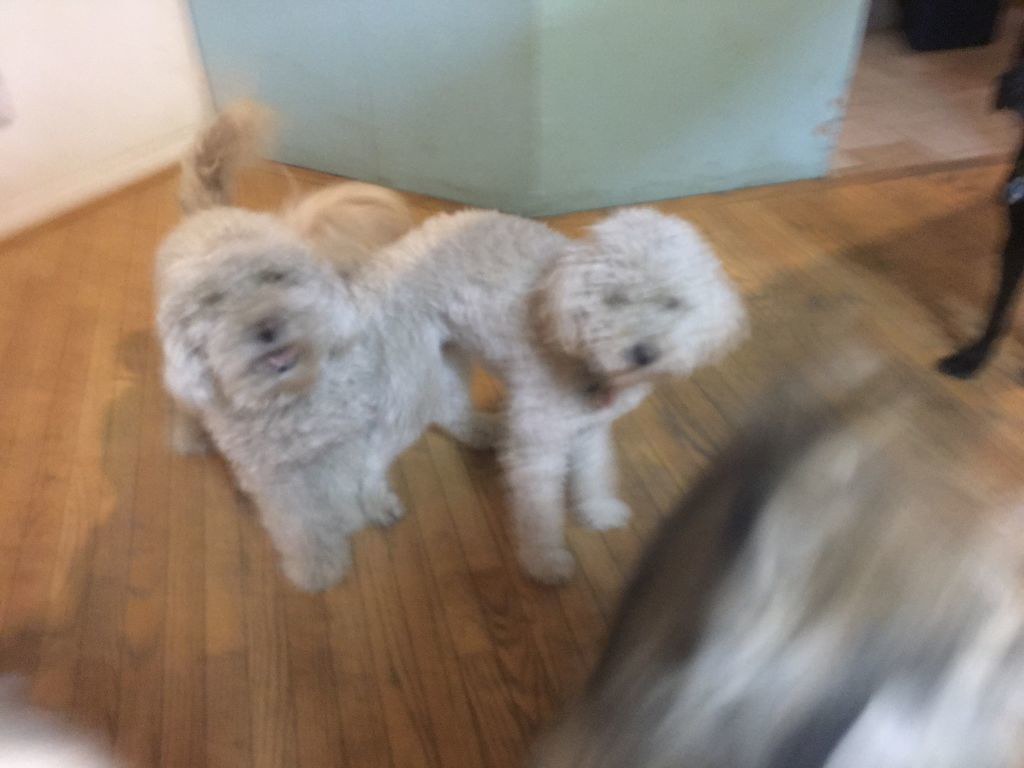This somewhat blurry photograph captures two beige, curly-haired dogs resembling poodles, standing side by side on a hardwood floor in a domestic setting. Both dogs are attentively looking at the camera, one panting with an almost smiling expression while the other keeps its mouth closed. Their tails appear to be wagging excitedly. The dogs are framed by a blue wall that transitions into a white wall at the corner, adding depth to the background. A chair leg is visible on the right side of the image, and the upper right corner reveals a glimpse of a tiled white floor, possibly leading into a kitchen. Additionally, the lower right corner shows the blurred back of someone's head, possibly the person taking the photo, and an indistinct cushion or couch side at the forefront of the frame.